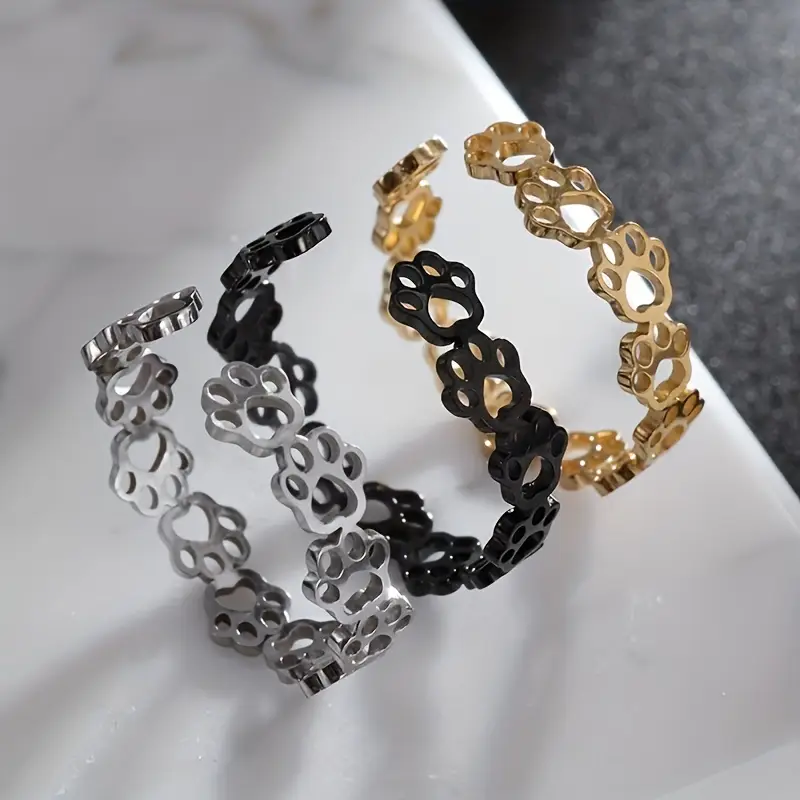This professionally captured, close-up image showcases a trio of metallic bracelets designed with repeated paw print patterns. Each bracelet is composed of interconnected, open-work dog paw prints that arc to form a circular shape, flexible enough to fit around the wrist, suggesting their appeal to pet lovers. The bracelets are presented in three distinct colors: silver, black, and gold, arranged diagonally from the middle left to the upper right portion of the image. They rest on a sleek, white surface with a hint of a gray marbled background, which, although slightly blurred, adds depth to the composition. The high-quality lighting and focus suggest that this image is likely intended for a professional catalog or advertisement.